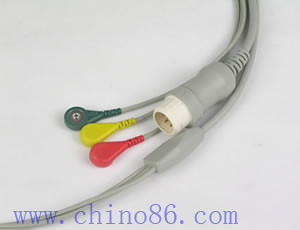The image showcases a specialized gray cable for medical equipment, most likely designed for an EKG machine, given its multiple adapter ends and colored leads. The primary cable branches out into three subsections: the first splits into three distinct colored leads—red, yellow, and a dark green or blue, which appear to be electrode attachments. The second branch features a large multi-pin plug commonly used for interfacing with devices. The third branch, which splits into three as well, is partially obscured and its connectors are not visible. The entire assembly is set against a clean white background with the website "www.chino86.com" displayed in blue, typewriter-style font at the bottom, possibly indicating the product's manufacturer or retailer.